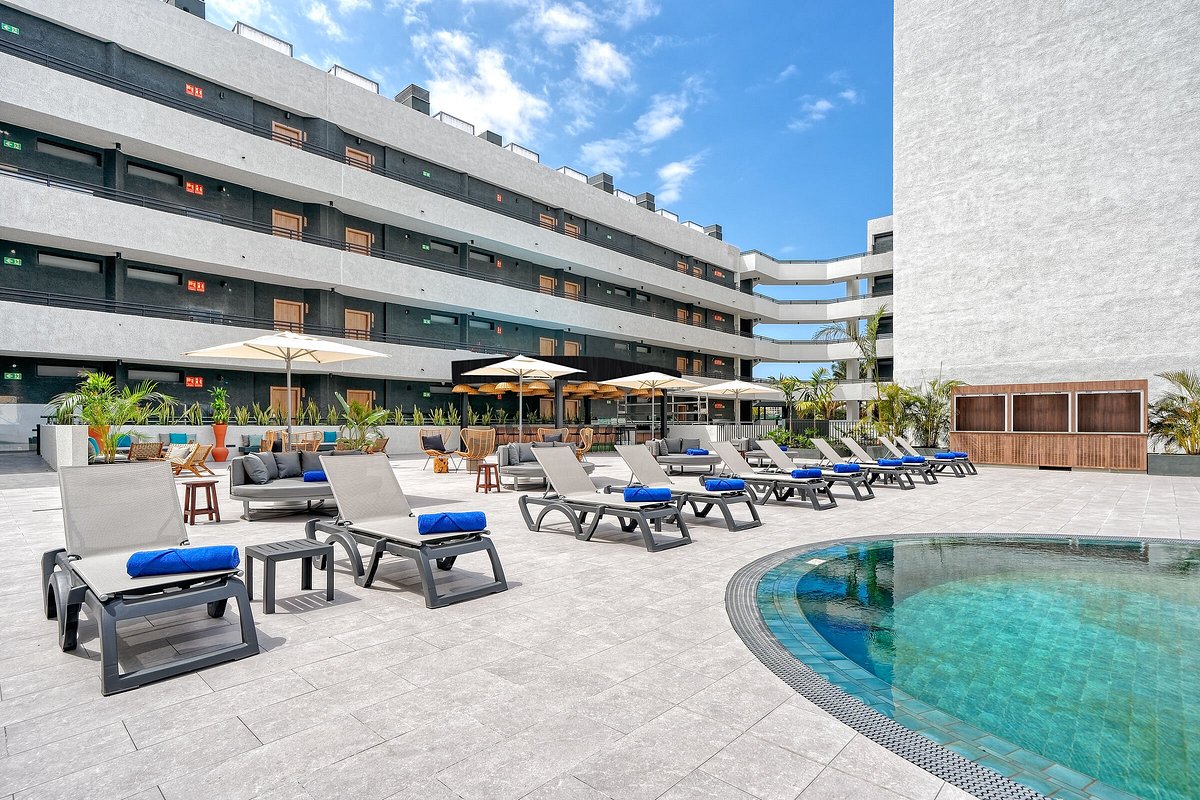This photograph captures an outdoor scene featuring a multi-level building that appears to be a hotel or beach stay area. The building on the left side of the image is four stories tall, with black and grey walls and an upper deck on the roof. Each level of the building has numerous doors and black accents on the walkways in front of the rooms. There are connecting walkways that lead to another taller building, also grey in color.

In the surrounding area, the ground is grey cement. There are multiple chairs scattered around, each with a blue bag, and additional furniture like couches and wooden stools. On the right side of the area, there's a pool surrounded by pool chairs. The scene includes tropical trees and plants with green leaves, adding a touch of nature to the setting. The sky above is a clear blue with some white clouds.